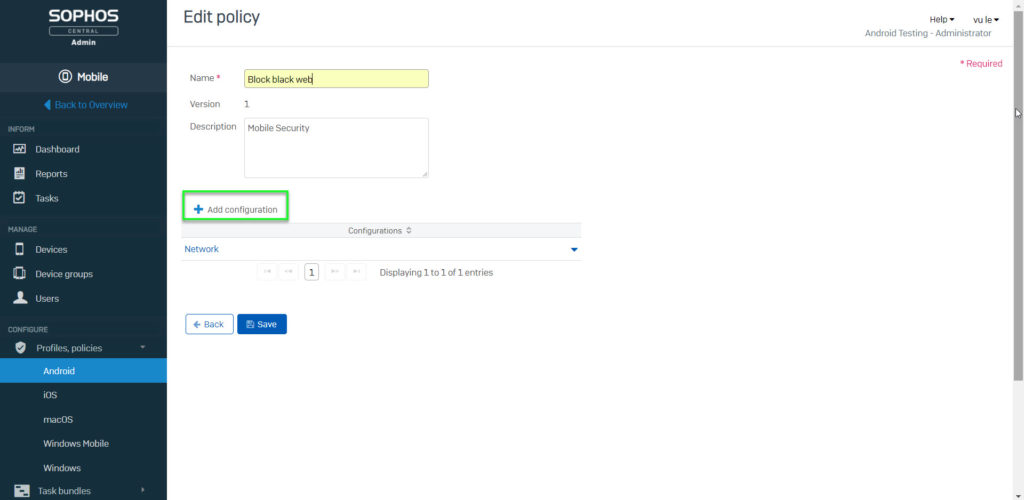Screenshot of the Sapphos website interface:

The screenshot shows the left sidebar, the main editing panel in the center, and some administrative details on the right.

**Left Sidebar:**
- **Theme:** Blue background with white lettering.
- **Top Section:** 
  - The word "Sapphos" is prominently displayed.
  - Inside a small box, the word "Central" is written, followed by "Admin."
  - An icon of a mobile phone is displayed next to the word "Mobile."
  - Below this, in blue lettering, it says "Back to Overview."

- **Inform Section:**
  - "Dashboard" with an icon.
  - "Reports" with an icon.
  - "Tasks" with an icon.

- **Manage Section:**
  - The header reads "Manage."
  - Lists "Devices," "Device Groups," and "Users," each with their corresponding icons.

- **Configure Section:** 
  - The header is "Configure" and the list includes:
    - "Policies"
    - "Profiles"
    - "Android"
    - "iOS"
    - "Mac OS"
    - "Windows Mobile"
    - "Windows"
    - "Task Bundles"

**Main Editing Panel:**
- The title "Edit Policy" is displayed.
- There's a text box labeled "Name," containing the text "Block black web." The text box has black lettering on a yellow background.
- The word "Version" is displayed underneath, with the version number "1."
- Further down, a large text box labeled "Description" contains the words "Mobile Security."
- Below the description, there is a green box with "Add Configuration" written inside it next to a blue plus sign.
- The section "Configurations" shows the status "Network displaying 1 of 1 of 1 entries."
- At the bottom, there are "Back" and "Save" buttons.

**Right Sidebar:**
- The section reads "Android Testing - Administrator."

This descriptive caption provides a thorough breakdown of the elements visible in the screenshot, allowing for a clear understanding of the Sapphos website interface.